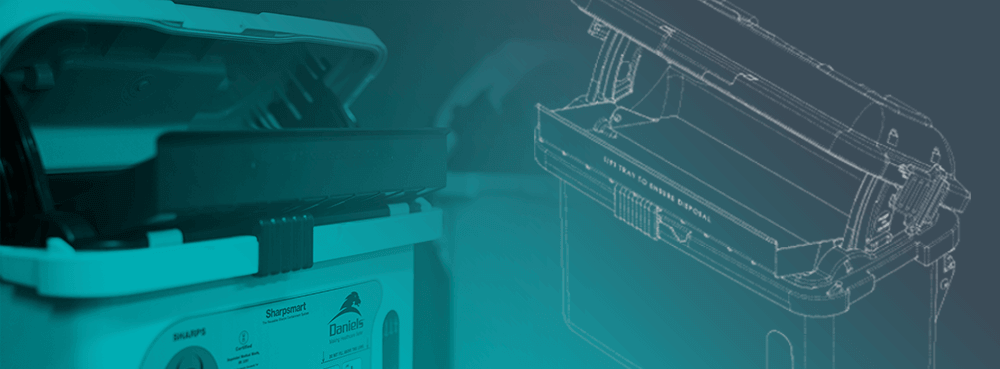The image is a horizontally rectangular photograph, predominantly tinted in blue shades, suggesting unique lighting or underwater settings. The setting is indoors. On the left side of the image, there's a white container with a grey lid that is open, revealing a black tray inside. The container bears the label "Shop Smart Daniels," and although partially blurred, the word "deposit" can be seen on the edge. The background behind the container is dark green. On the right, there is a graphic print, yellowish in color, of the same container, resembling a mechanical drawing. Both images are captured against a blue and partially grey background. Some small, unreadable text is also present in the graphic print. The overall scene is detailed with sharp contrasts between the photographic and drawn elements, providing a comprehensive view of the container.